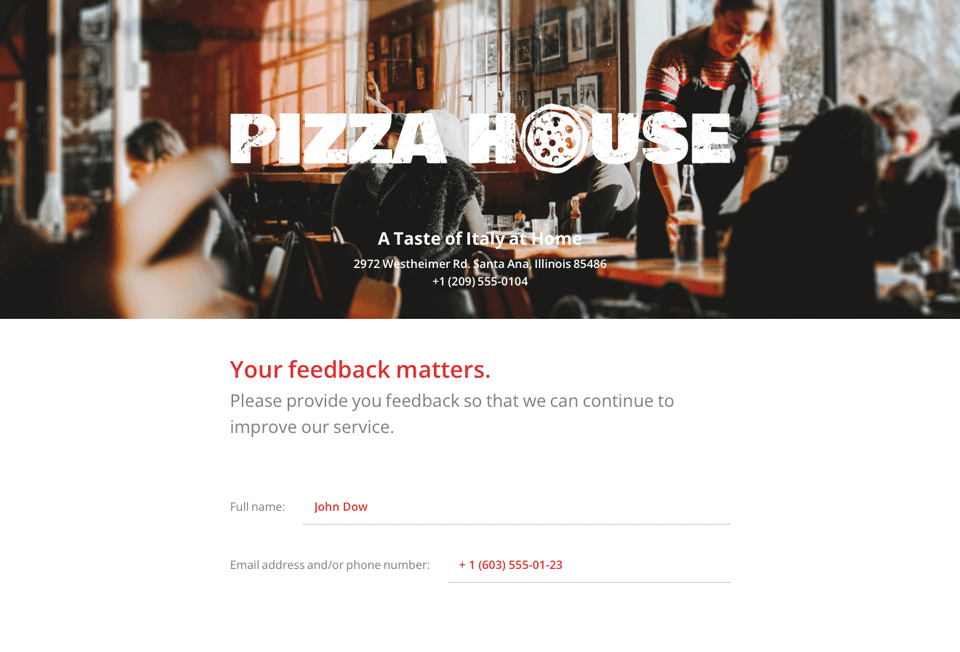The screenshot captures the homepage of a restaurant or food delivery service named "Pizza House." The upper half features a vibrant photograph of the restaurant's interior, showcasing several tables, numerous framed photos adorning the walls, and large windows with curtains allowing ample natural light to flood the space. A female server, dressed in a black apron and a striped top, is visible, adding a welcoming touch to the scene. Dominating the top of the image is the restaurant's name, "PIZZA HOUSE," in bold white capital letters, with the 'O' cleverly replaced by a pizza icon. 

Beneath the restaurant's name, the tagline "A Taste of Italy at Home" is prominently displayed, followed by the address, "2972 Westheimer Road, Santa Ana, Illinois 85486," and the phone number, "1209-555-0104," all in white text.

The lower section of the image, set against a white background, features a customer feedback form. In bold red letters, it states, "Your Feedback Matters." Below this, in gray text, a prompt encourages visitors: "Please provide your feedback so that we can continue to improve our service." The form includes two gray text fields labeled "Full Name" and "Email Address and/or Phone Number," both of which are filled in with red, awaiting user input.